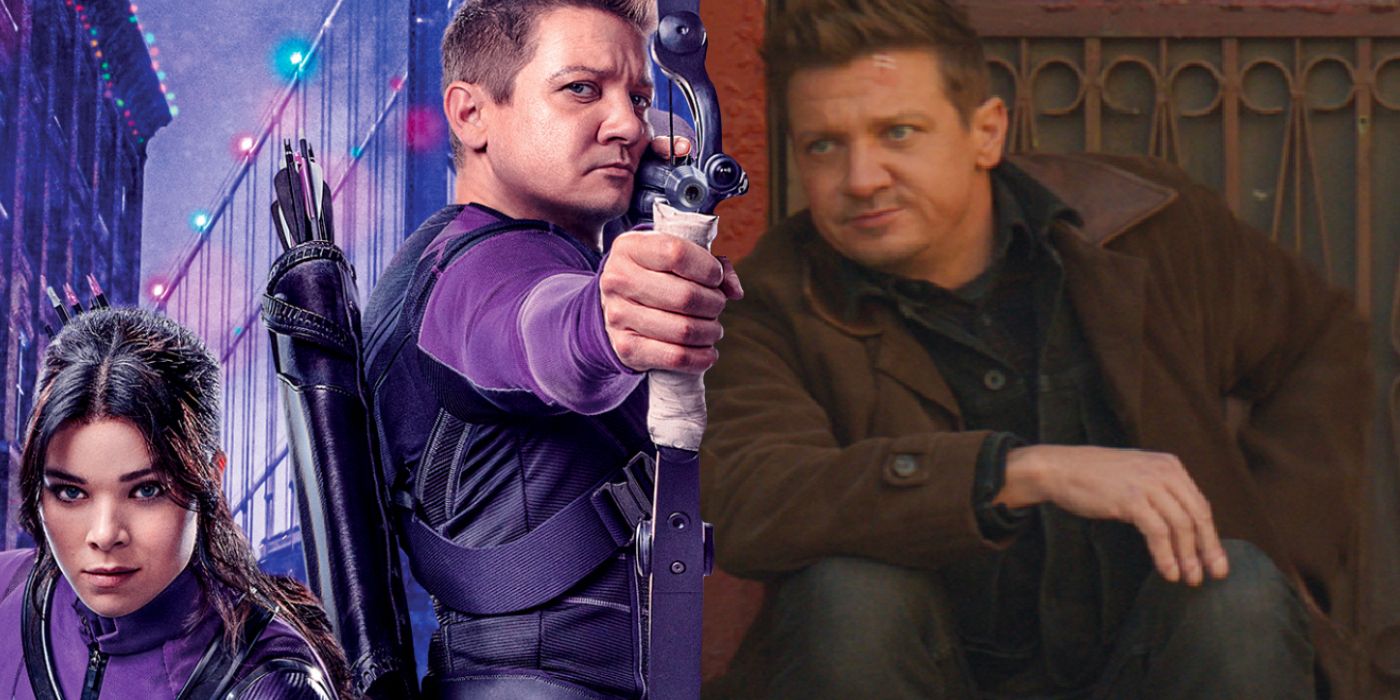This image features two juxtaposed scenes of actor Jeremy Renner. On the left, a stylized depiction places him in a high-tech, superhero persona, fully equipped with a sophisticated bow and quiver filled with arrows. Renner, portrayed with a serious demeanor, stands poised to shoot, his bow directed towards the viewer. He dons a purple shirt under a black vest, complemented by a woman crouching nearby in a matching purple jumpsuit, indicating a possible collaboration. The background depicts a dramatic purple sky with a suspension bridge adorned with green and red lights, alongside a looming building. To the right, a contrasting, realistic image of Renner is set in a more grounded scenario; he sits casually on a step, dressed in a brown corduroy jacket over a black and gray plaid shirt, paired with jeans. Behind him is a textured door with designs, suggesting an urban setting. This dual portrayal underscores his role in a popular series, likely recognized by fans.